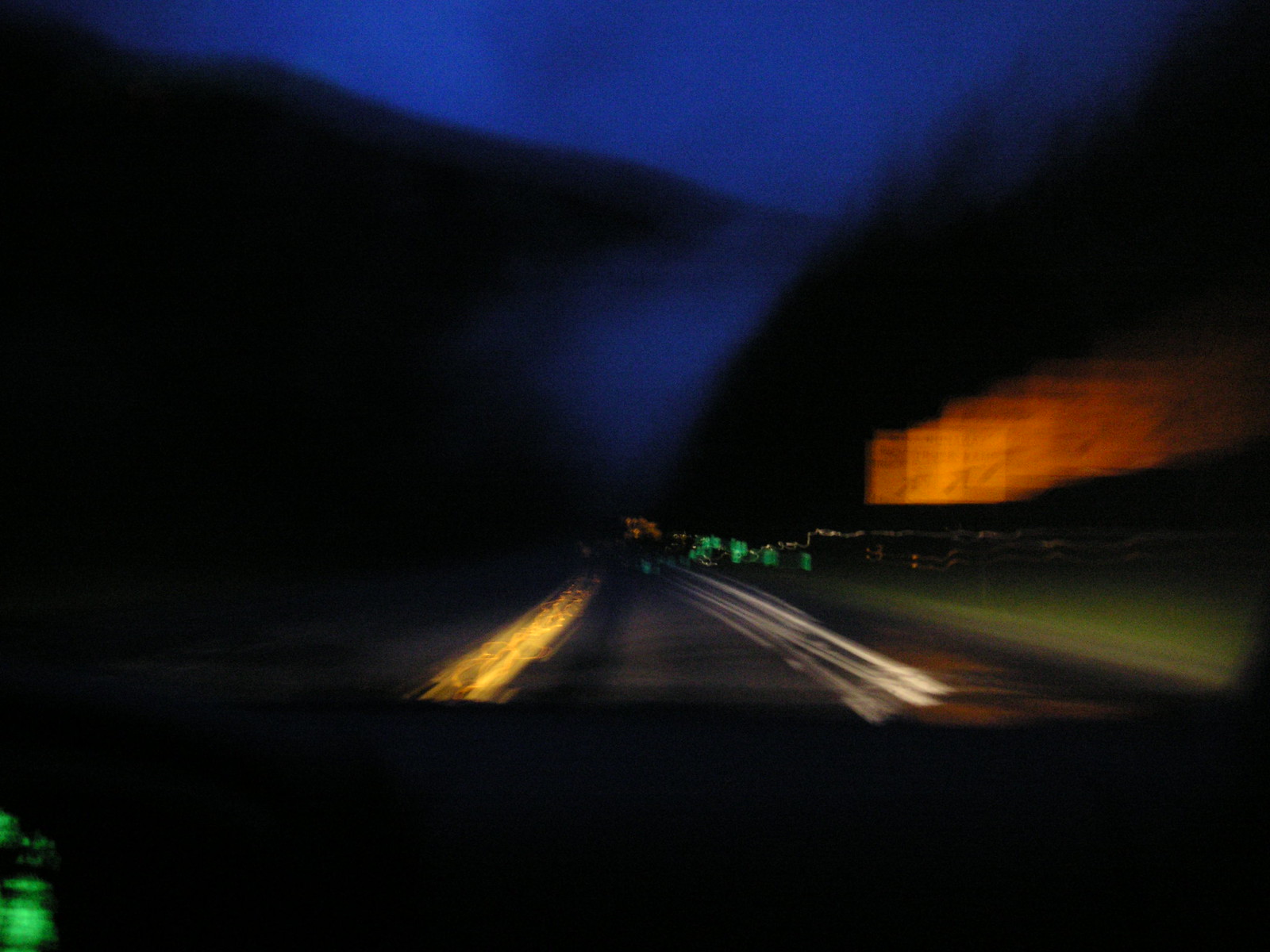The image captures a driver's perspective through a windshield at night. At the bottom of the frame, there is significant blackness, suggesting the dashboard. To the left, a slightly visible green element, likely the speedometer, shows faintly. The road ahead stretches into the distance with a dark sky above, transitioning from black to dark blue and back to black. On the roadside, green barrels, fencing, flags, and patches of grass are discernible. A series of signs, blurred into streaks of orange, yellow, and black, indicate the vehicle's movement. In the distance, a few blurred lights mark the continuation of the road.